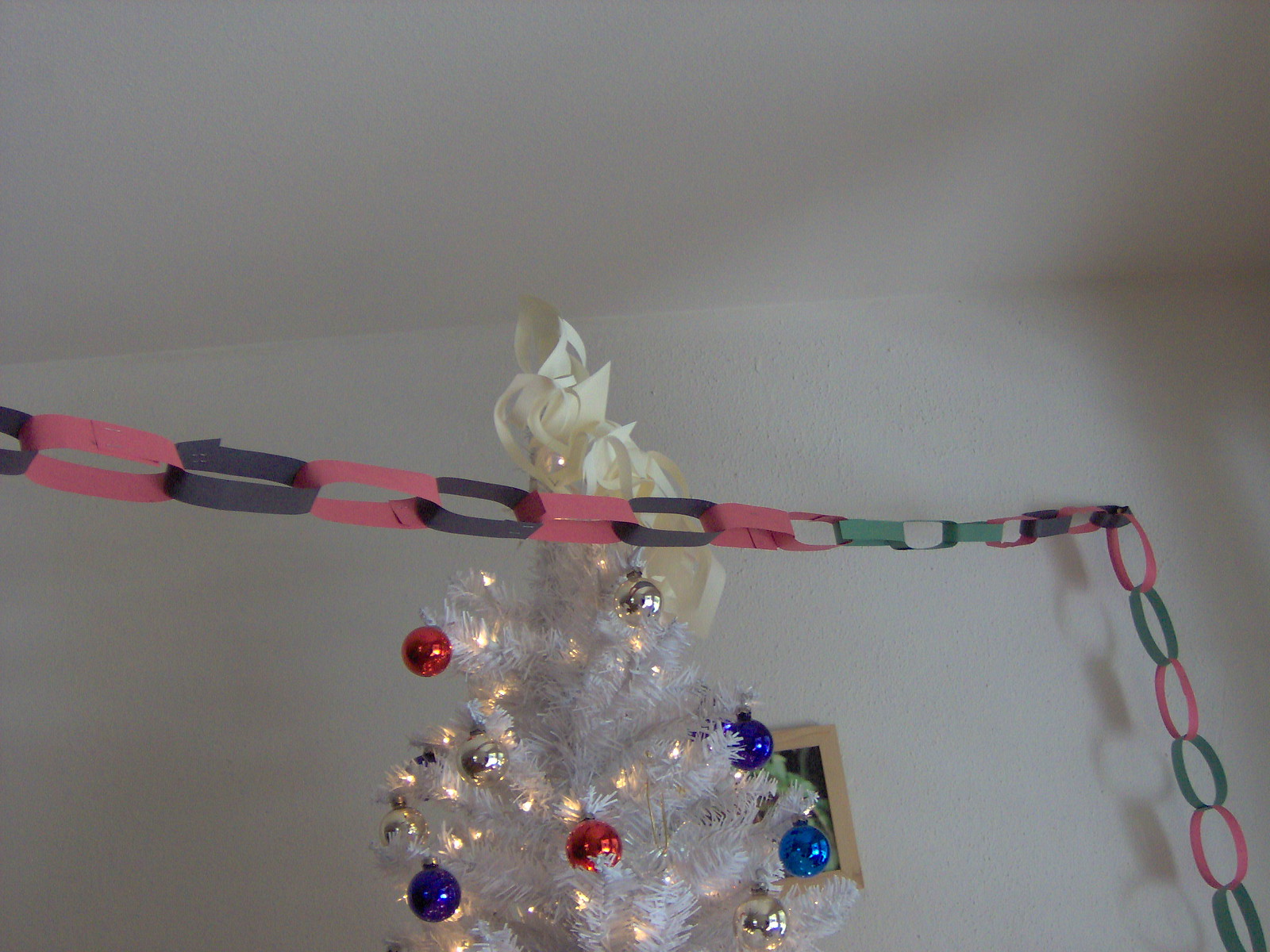This vertical, rectangular color photograph, taken inside a dimly lit room with standard white drywall, captures a festive holiday scene. Dominating the image is an artificial white Christmas tree adorned with a white geometric star tree topper and bright yellow-white string lights. The tree is decorated with an assortment of ornaments, notably blue and red bulbs, along with a single gold bulb. Adding a playful, nostalgic touch, a large, colorful paper chain is strung in front of the tree, presumably made as a Christmas countdown decoration. The chain features alternating red and black loops, hanging down along the right side of the tree, contrasting with a few additional purple, orange, and green loops. A partially obscured wall decoration can be faintly seen behind the tree, adding to the cozy indoor setting. The subdued lighting casts various shadows, enhancing the intimate, homey atmosphere of the scene.